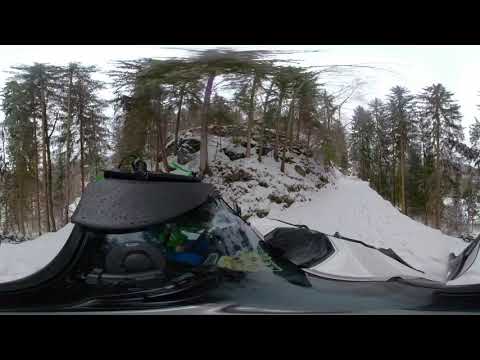This image captures a winter scene dominated by tall, thin trees with sparse green leaves standing on a mound of snow interspersed with rocks, all under a stark white sky. The scene appears slightly warped, giving a wavy effect to the right side. In the foreground, a black snow vehicle is prominent, likely moving forward. It features a large, shiny, glassy instrument protruding from its hood, likely a camera reflecting the snowy surroundings. The vehicle's bed and components glisten as they catch the light, adding to the wintery feel. The path ahead is blanketed in snow, leading up a hill flanked by tree lines and scattered rocks. The atmosphere suggests a remote, mountainous area.